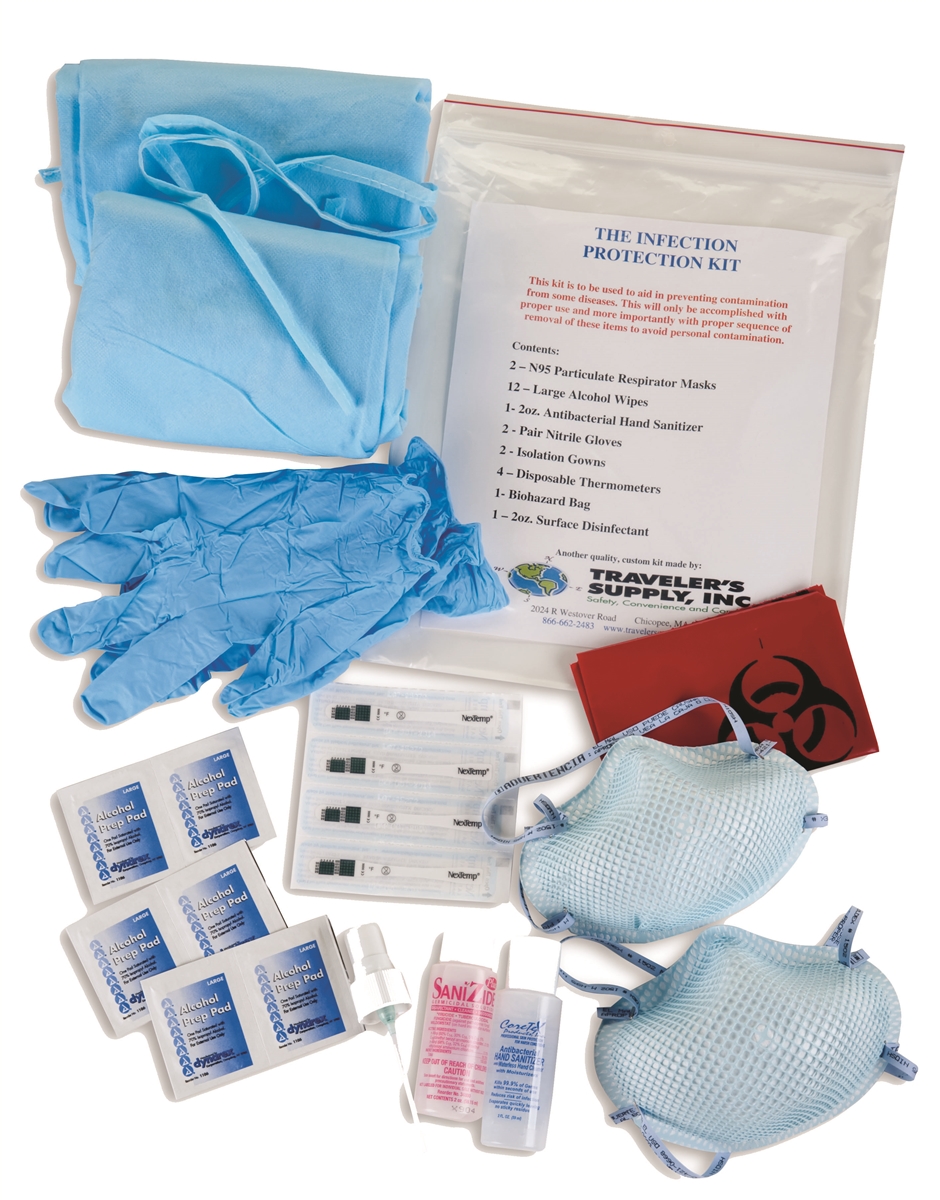This is a detailed bird's eye view of an infection protection kit laid out against a completely white background. In the top left corner, there is a neatly folded pair of blue scrubs. Directly beneath the scrubs, crumpled blue nitrile gloves are visible. To the right of the gloves is a plastic clear bag containing the infection protection kit, which features an info sheet detailing its contents in blue, red, and black colored fonts. Below the infection protection kit is a vibrant red biohazard bag emblazoned with a black biohazard symbol. Positioned under the biohazard bag are two disposable face masks. To the left of the masks, several COVID test strips are arranged in a clear paper package. In the center bottom, there are two distinct bottles of liquid—one red and the other blue, identified as a two-ounce surface disinfectant and hand sanitizer—along with a pack of large alcohol prep pads in a white and blue package. Lastly, at the very bottom left, there is a pack of additional alcohol wipes arranged in blue packaging.